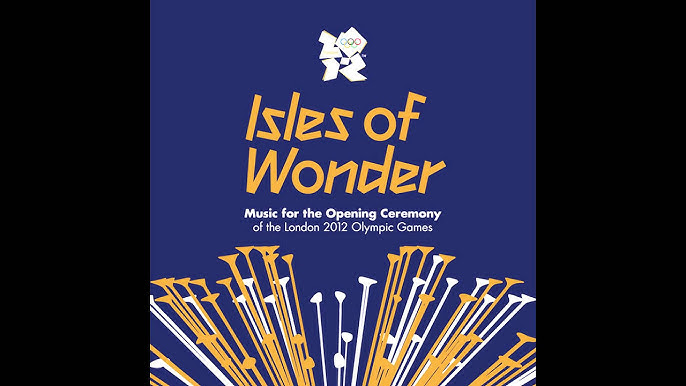The image is an advertisement poster for the London 2012 Olympic Games. It features a bold, slanted blocky font with the text "Isles of Wonder" prominently displayed in yellow. Beneath this, in smaller white text, it reads, "Music for the Opening Ceremony of the London 2012 Olympic Games." The background is navy blue with black borders on either side. At the top center of the poster, there is a small Olympic logo, creatively designed in the shape of "2020," with the five iconic Olympic rings embedded in the zero, each ring in its traditional color. Below the text, a series of thin, trumpet-like instruments in alternating yellow and white extend outward in various directions, creating a dynamic, fan-like pattern. The overall composition of the poster brilliantly captures the essence and excitement of the event.